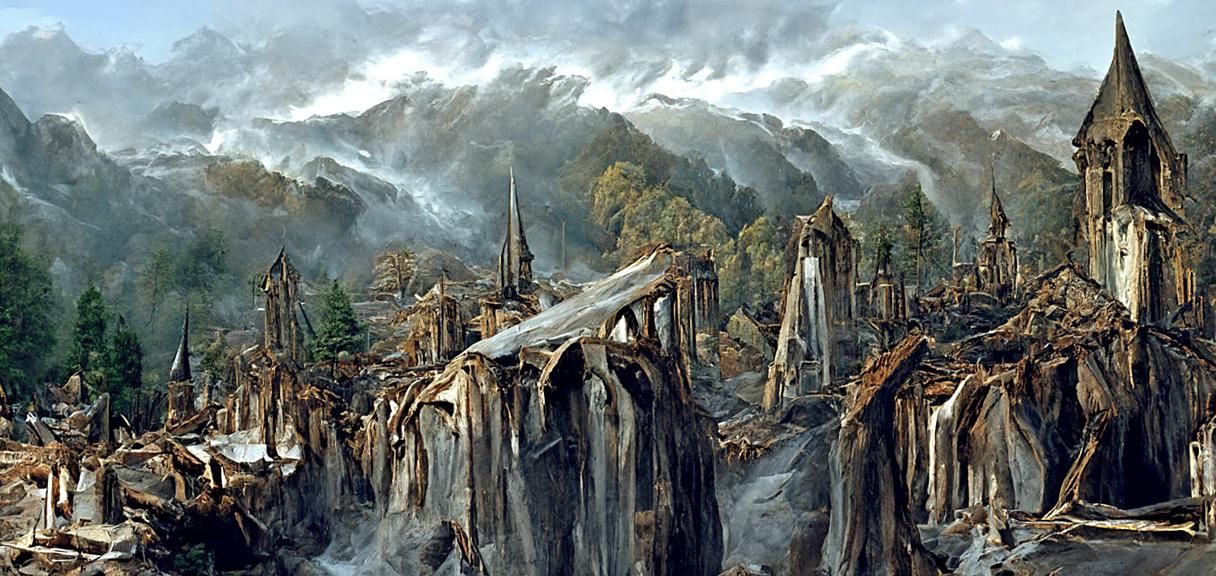The image is a detailed and surreal illustration of a desolate landscape, reminiscent of a scene from Rivendell in Lord of the Rings. Dominated by a foreboding atmosphere, the scene features dark, burnt-down trees in the foreground, their tops appearing melted and shattered, starkly contrasting against the remnants of a village or ancient buildings in various states of disrepair. The structures, which have an eerie, church-like appearance with warped and bending steeples, stand amidst a zone of destruction, suggesting they have been ravaged by fire. Spanning from the bottom left to the top right, a forest strip adds to the bleak panorama with hues ranging from dark green to gray-green. Towering over the scene, mist-covered hills with dark gray and green slopes merge into a gray-blue sky, where the peaks are obscured by a white veil, possibly snow or fog, enhancing the ethereal and somber mood of the setting.